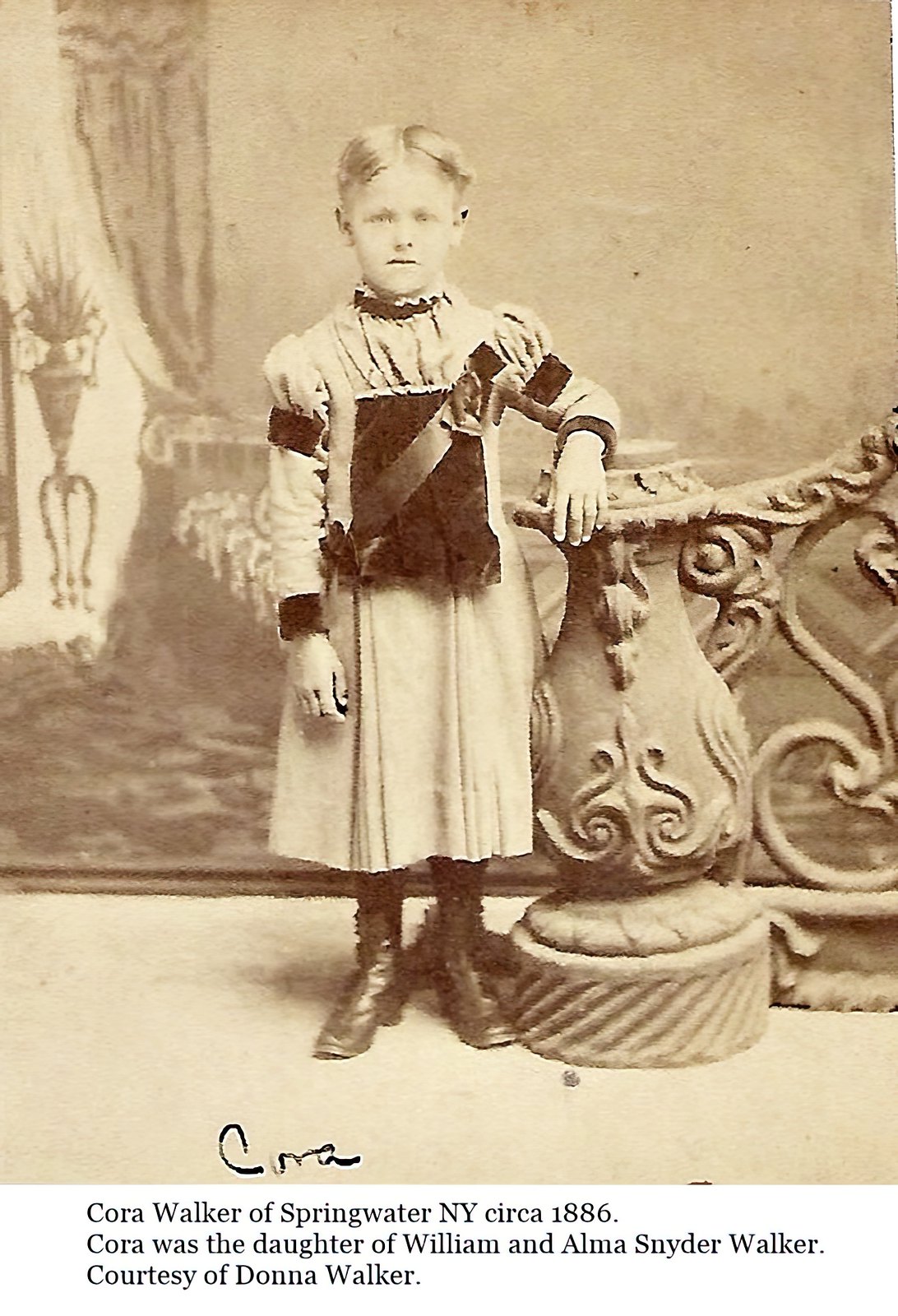This black and white photograph, approximately six inches high and four inches wide, depicts a young girl named Cora Walker, posing indoors against an ornate vase or stone pedestal. The photograph, taken circa 1886, shows Cora wearing a long dress-like garment with puffed shoulders and dark narrow sleeves. Her short hair is neatly parted in the middle, and she gazes directly at the camera with a solemn expression, her left arm resting on the pedestal while her right arm hangs by her side. The setting features an old photographer's backdrop, likely a painted image of a room, with a pale cream-colored floor occupying the bottom third of the picture. Inscribed in black ink at the bottom is her name, "Cora," along with typeset text that reads: "Cora Walker of Springwater, New York, circa 1886. Cora was the daughter of William and Alma Snyder Walker. Courtesy of Donna Walker."